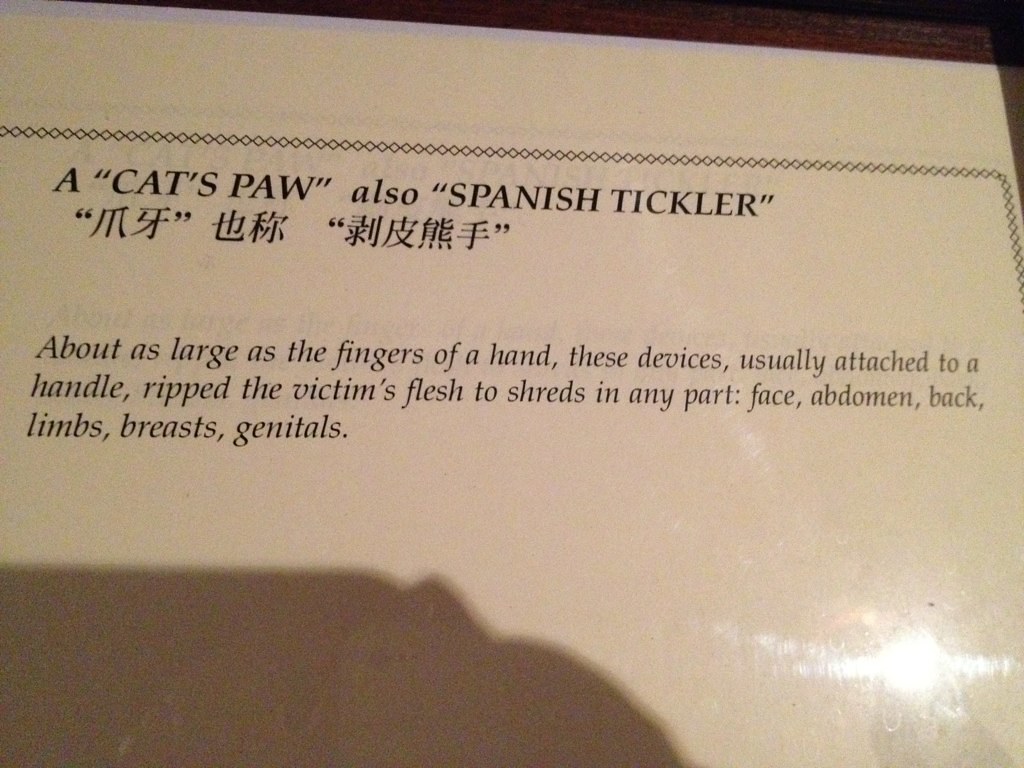The image captures a light gray mat with a diamond-patterned border, intricately designed around the text. The mat lies on a wooden surface, visible only as a slight sliver in the upper right corner. The main text on the mat, enclosed in double quotations, reads "A cat's paw, also Spanish tickler." Directly beneath this, there is a translation in Chinese characters, followed by a paragraph in smaller, italicized text. This paragraph details the gruesome nature of the device, stating, "About as large as the fingers of a hand, these devices, usually attached to a handle, ripped the victim's flesh to shreds in any part: face, abdomen, back, limbs, breasts, genitals." At the bottom of the image, light illuminates the paper, casting a shadow on the lower left side, which might suggest the presence of the person taking the picture.